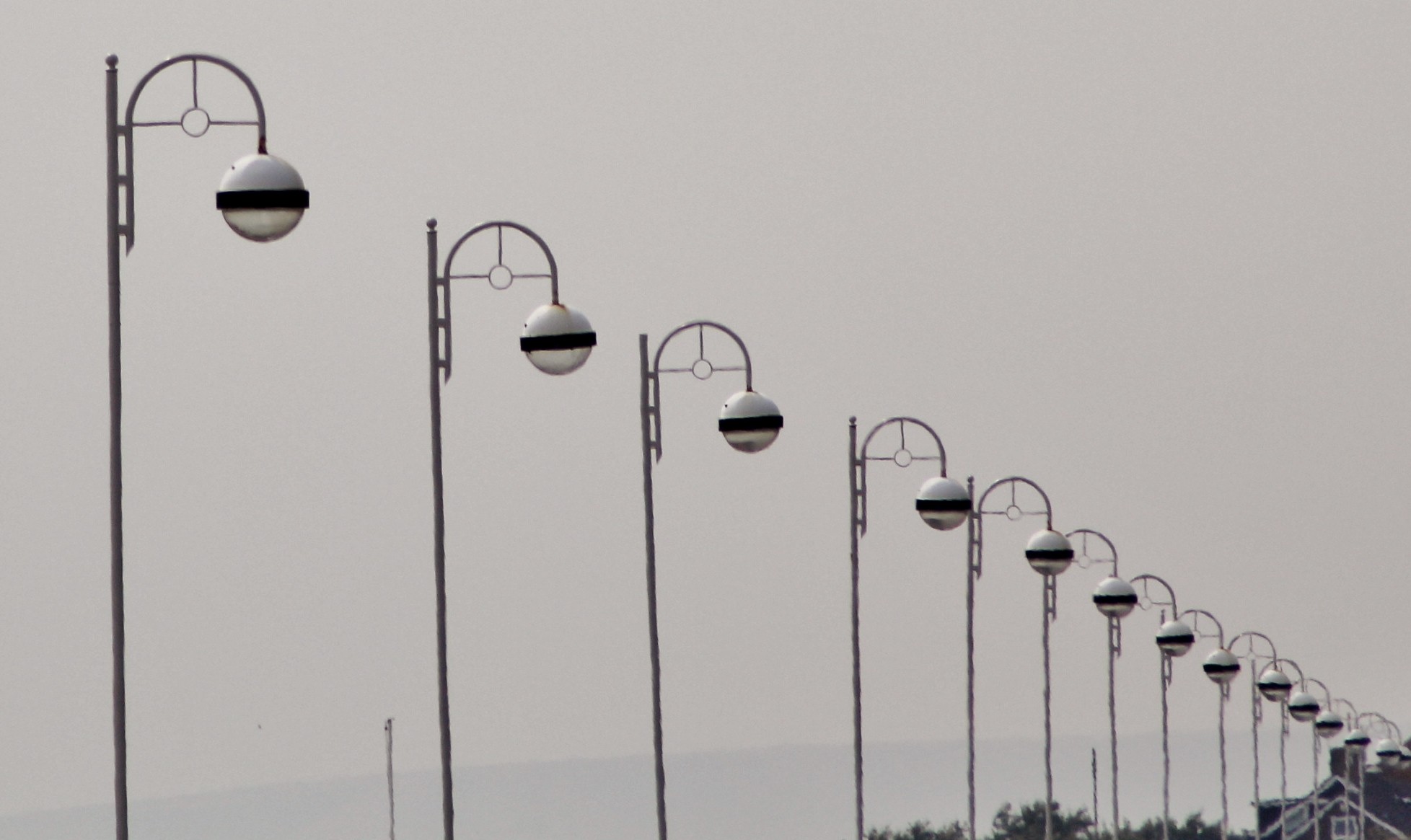This photograph captures a line of approximately 16 or 17 identical street lamps on an overcast day. The image is taken from ground level, looking upwards and across the length of the lamps, creating an optical illusion where the lamps appear to get smaller as they recede into the distance. Each tall metal pole supports an upside-down U-shaped arm that curves up and down, culminating in a rounded, white-topped lamp with a black band around its center, and a large glass bulb at the bottom. The lampposts, seemingly spaced five to ten feet apart, stretch out diagonally across the image, creating a repetitive pattern that draws the eye towards the horizon. The background features a gray, smoggy sky with a faint mountain skyline in the distance. A house is partially visible at the bottom right corner, and the ocean edges the horizon, adding depth to the composition. None of the lights are turned on, enhancing the somber, overcast ambiance of the scene.